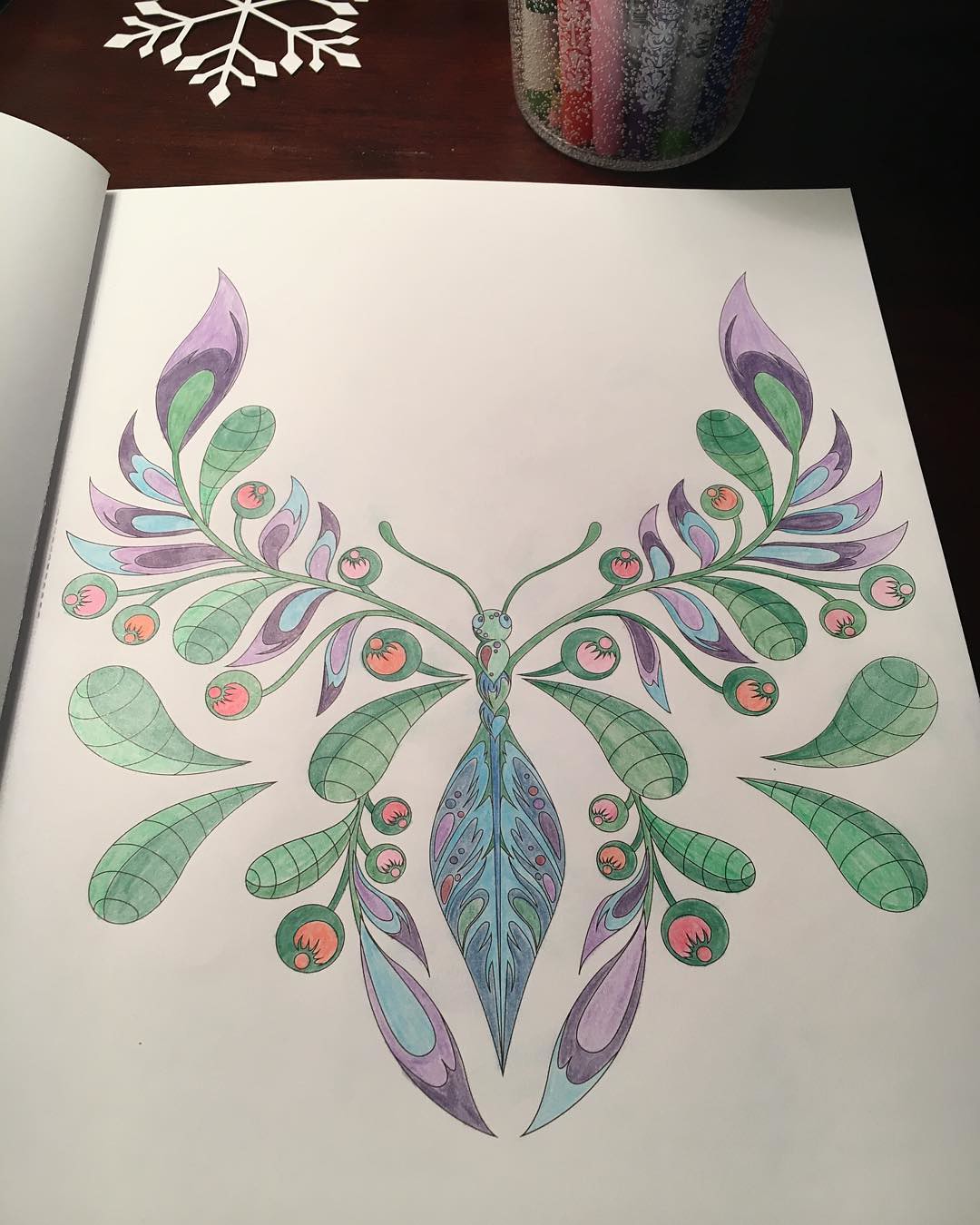In this detailed sketch, the focal point is an insect-like figure situated centrally, characterized by green antennas and a small, circular green head and body. The creature's abdomen transitions into a blue leaf adorned with various intricate colors. Extending from the central figure are two prominent vines, each decorated with a mixture of leaves in green, purple, pink, and blue hues. To the lower left of the sketch, a cluster of green leaves begins to emerge, while above these, additional leaves form in bulbous, circular shapes, showcasing red and green interiors. Further down, the design incorporates light blue, purple, and pink leaves, adding depth and variety to the composition.

The entire drawing is executed on a gray piece of paper, providing a neutral background that highlights the vivid colors of the sketch. In the top left corner of the artwork, a white snowflake design is visible, adding a touch of contrast and texture. To the right of the snowflake, the bottom portion of a container filled with utensils can be seen, and the rest of the background is predominantly white, ensuring that the intricate details of the sketch stand out prominently.